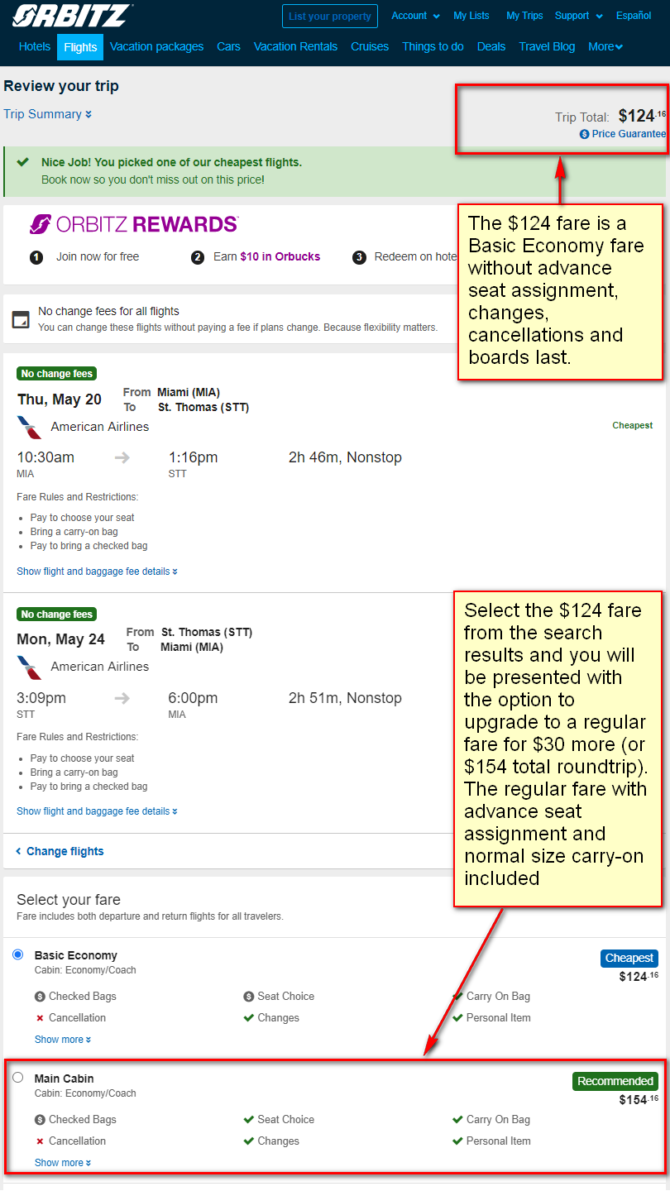The image depicts a travel booking website with a detailed interface primarily in navy blue, gray, white, and green colors.

At the top, there's a navy blue banner featuring the word "Orbits" in bold white text. Centrally placed below this, there's a rectangular border with the option "List your property" in blue text. Next to it are additional options: "Account" with a drop-down menu, "My List," "My Trips," "Support" with a drop-down, and an option for "Español."

Further down, under the "Orbits" banner, there's a navigation bar with various categories: "Hotels," "Flights" (highlighted with a medium blue background and white text), "Vacation packages," "Cars," "Vacation rentals," "Cruises," "Things to do," "Deals," "Travel Blog," and "More" with a drop-down menu.

The subsequent section has a gray background and contains trip review details. It includes a "Review your trip" header and a "Trip summary" followed by details within a red border, indicating a trip total cost of $124.16. There is mention of a price guarantee. Below this, a yellow box highlights that the $124 fare is a basic economy option without advanced seat assignment, changes, cancellations, and boards last. An arrow points upwards to the trip total.

A green background section praises the user with "Nice job! You picked one of our cheapest flights. Book now so you don't miss out on this price." Below this, a white banner promotes Orbits Rewards with a "Join now for free" offer, promising to earn "Orbucks" redeemable on hotels.

Another white banner states "No change fees for all flights." Immediately following this, there's a detailed white background section listing flight details:
- May 20th from Miami to St. Thomas via American Airlines.
- May 24th from St. Thomas to Miami, marked with "No change fees."

Below the flight details, options to change flights or select a fare are given, with "Basic Economy" being chosen (noted within a red border) and "Main Cabin" not chosen.

The detailed layout, multiple options, and highlighted sections make it easy for users to navigate and understand their booking choices on this travel website.